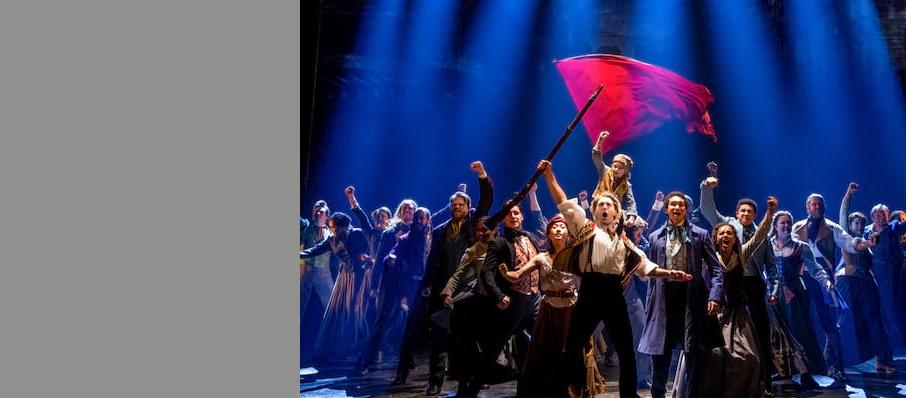The image depicts an elaborate scene from a Broadway musical, specifically "Les Misérables." On the right side of the image, a large blue block prominently displays the title "Les Miserables" in white text against the blue backdrop. The stage is filled with a large group of men and women, all dressed in period attire reminiscent of peasants from the 1800s, including petticoats, suspenders, and scarves. The performers, many of whom have longer hair and are adorned in old-timey clothing, appear intensely engaged in a dramatic and revolutionary tableau. A man in the center, dressed in a white shirt, dramatically holds a musket high above his head, while a red flag waves above the ensemble. The scene is bathed in dynamic lighting that enhances the theatrical atmosphere, with vibrant blue spotlights casting down from above. Many actors on stage have their fists raised and mouths open, likely mid-song or chant, conveying a fervent sense of uprising and defiance. Their exaggerated gestures and expressions contribute to the vivid and emotional portrayal of this iconic moment from the musical.